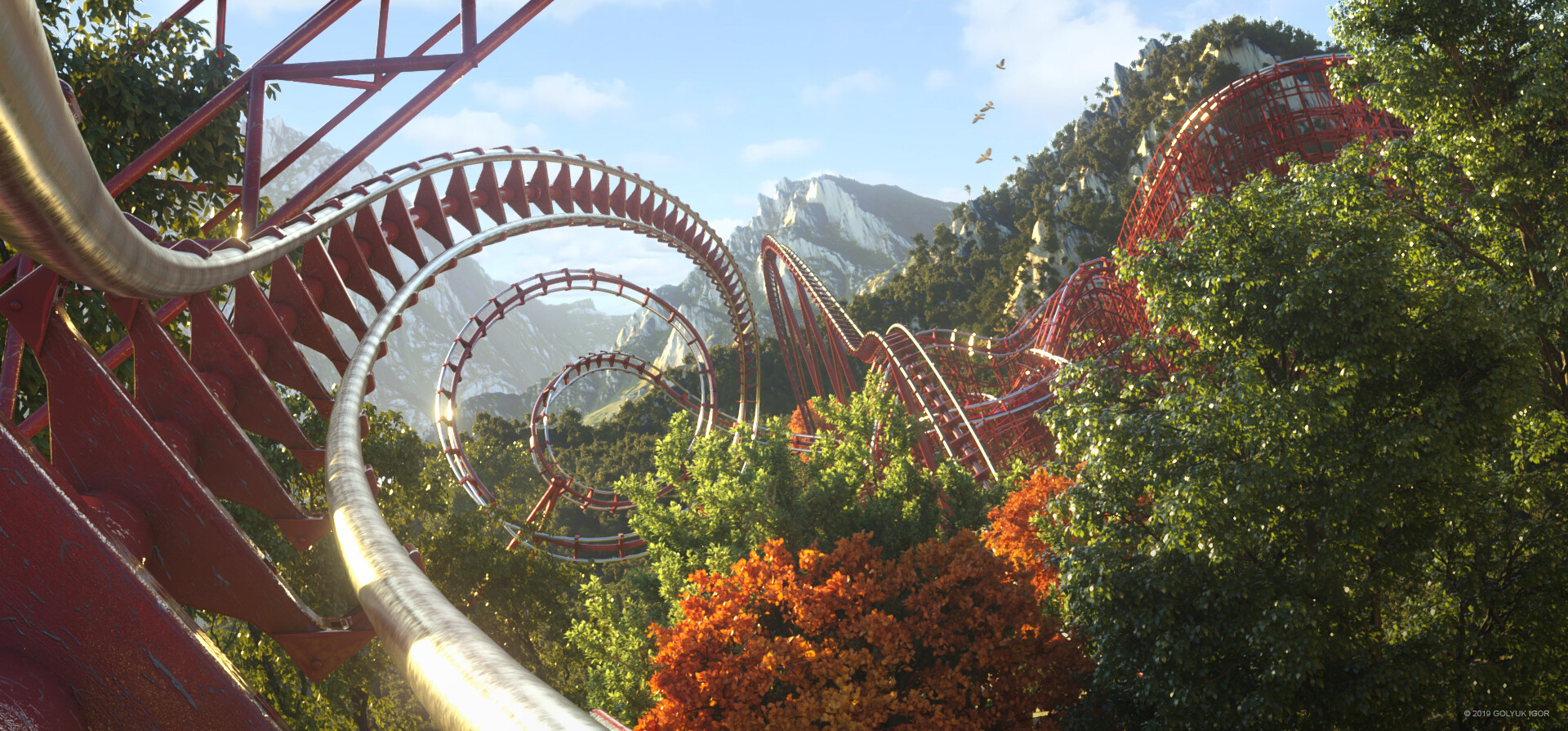The image depicts a detailed, computer-rendered roller coaster track stretching horizontally across a wide frame, with a lush, green forest and a prominent snow-capped mountain in the background under a vibrant blue sky dotted with puffy white clouds. From the vantage point within a carriage on the track, the coaster appears to start on the left-hand side with sleek silver rails and red triangular tracks, adorned with gold railing and white and red planks or dividers. The track initially heads to the right, entering a captivating spiral making three full rotations before transitioning into a sharp right turn. It then continues through a series of large, undulating hills and dips. The vibrant scene is interspersed with green treetops and a few orange leaves suggesting seasonal change. Birds, or perhaps bats, enhance the dynamic atmosphere, flying above the scenic landscape. The artistic rendering gives a sense of realism with its detailed textures and perspective, yet hints towards being a digital creation, possibly from a video game or an elaborate digital artwork.